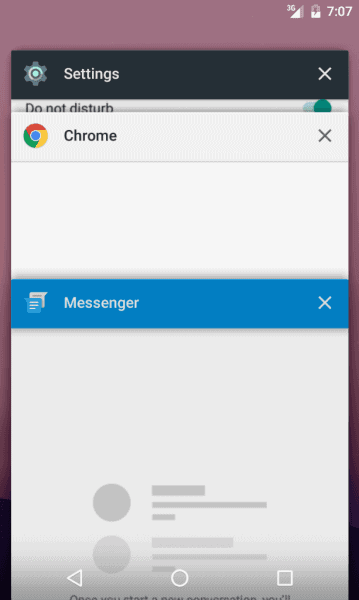In the image, someone has two different apps open on their device. The first app, Chrome, is visible below the settings. Chrome is the app currently being viewed, displaying the Messenger web interface. At the very top of the Chrome window, there is a header bar featuring the characteristic red, yellow, and green circular buttons on the left, allowing the user to minimize, maximize, or close the window. To the right side of the header, there is an option to exit the app.

Midway down the Chrome window, the word "Messenger" is written in white text, highlighted with a blue background. Below this label, the interface shows two rectangular sections, each of the same size, but one is in a darker shade of gray while the other is lighter. These sections likely represent different message threads or options.

At the bottom of the screen, there are three navigation buttons: a back button, a circular home button, and a square multitasking button. Above the Chrome window, part of the device's settings is visible. The settings section, featuring a gear icon on the left and the word "Settings" in white text, is partially obscured but still identifiable. There is an X button within the settings interface, indicating an option to close it.

Just below the settings section, the "Do Not Disturb" option is faintly visible at the top right. The top right also shows the device is connected to a 3G network, the battery is charging, and the current time is 7:07. The background color seen around the edges of the apps is a brownish-pink hue. The Chrome interface itself is displayed with a white background, contrasting with the black banner at the very top that hosts the other elements like network status and time.